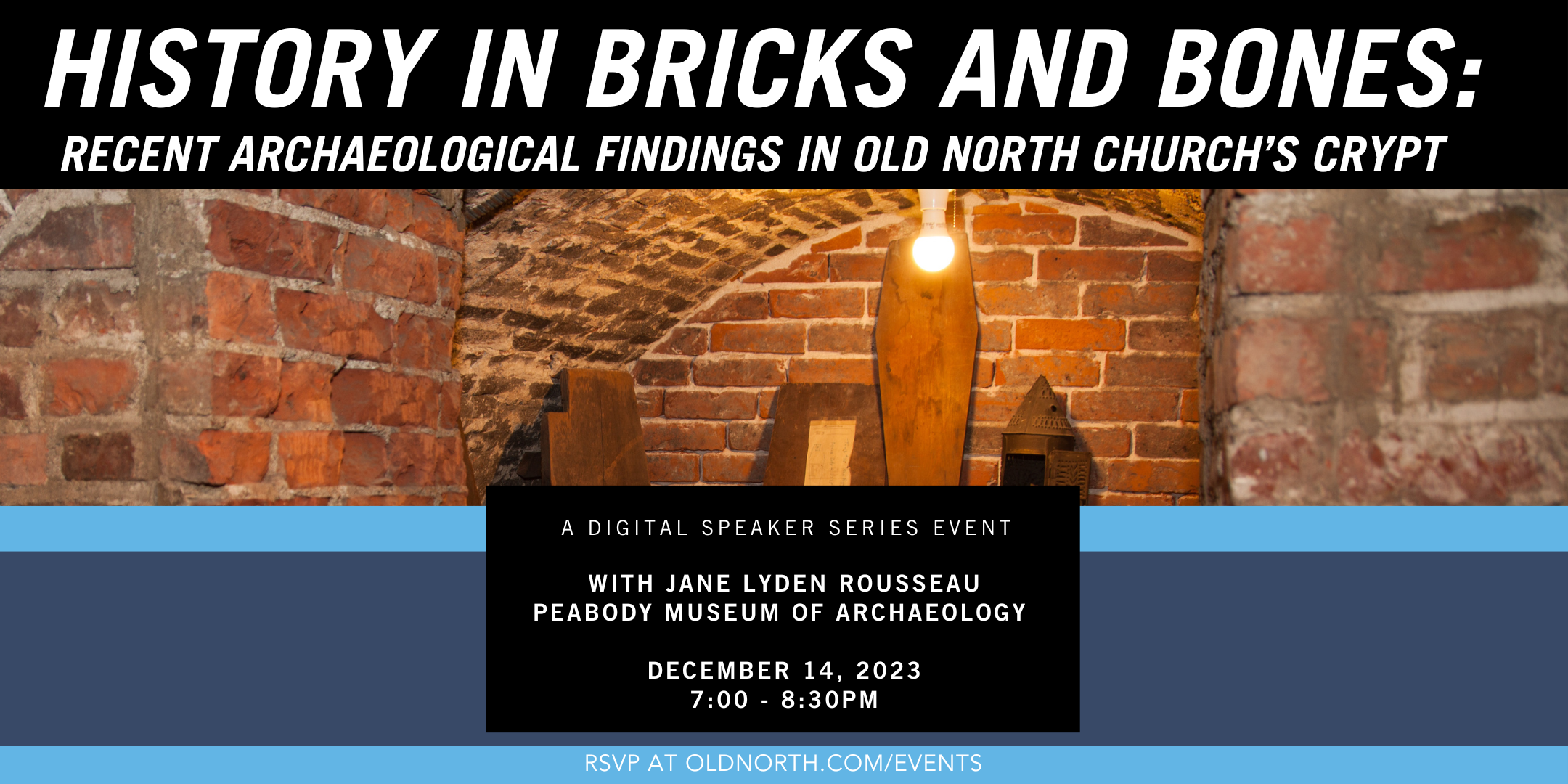The event advertisement image, titled "History in Bricks and Bones: Recent Archaeological Findings in Old North Church's Crypt," features bold, all-capital white letters on a black background. Prominently displayed is a photograph of a historical brick structure's interior, possibly the basement of an old church, with archaic and weathered red brick walls forming a curved ceiling. The scene is dimly lit by a single lightbulb, revealing wooden coffins leaning against the walls, amplifying the sense of antiquity. The bricks appear aged, dirty, and slightly crumbly, enhancing the historic ambiance. Beneath this evocative image, the text details a digital speaker series event featuring Jane Linden Rousseau from the Peabody Museum of Archaeology, scheduled for December 14, 2023, from 7 to 8:30 PM. Attendees are instructed to RSVP at oldnorth.com/events. Color elements framing the text include a deep purplish-blue bar with light blue strips at the top and bottom, and a black rectangular box containing white text.